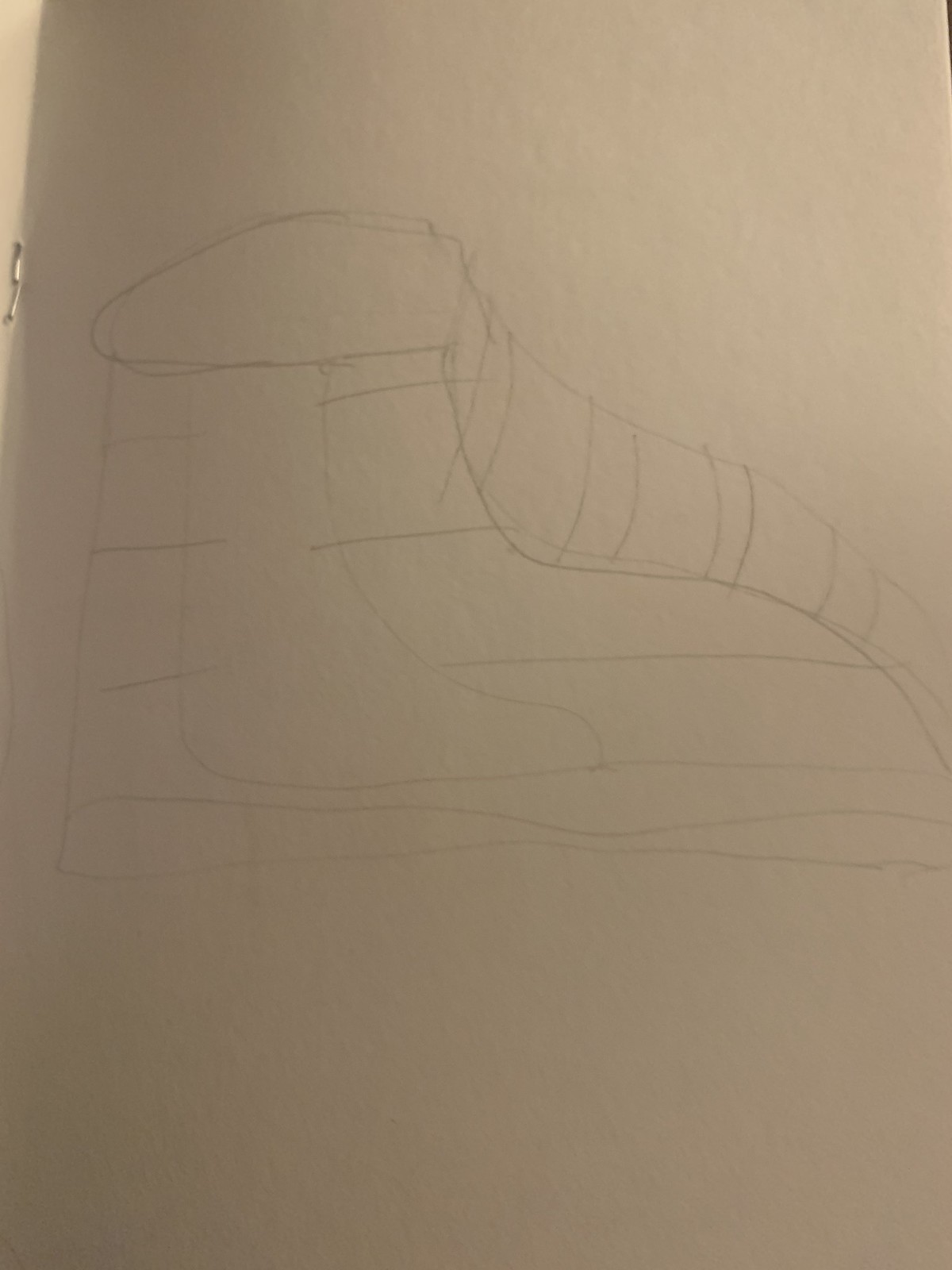A photograph captures a piece of paper featuring a pencil sketch. The paper is an off-white color and likely photographed in low lighting, resulting in a blurry, low-resolution image. The sketch appears to depict the side view outline of a shoe with a boxy, unconventional design. The drawing consists of numerous lines, with some sections darker and more defined, while others are faint and nearly blending into the paper. A visible staple is located on the left side of the paper, hinting at its attachment or previous use. Smudges and eraser marks are scattered across the sketch, indicating adjustments or corrections. At the top right corner of the image, a sliver of the dark background is visible, adding to the overall dim and shadowy ambiance of the photo.